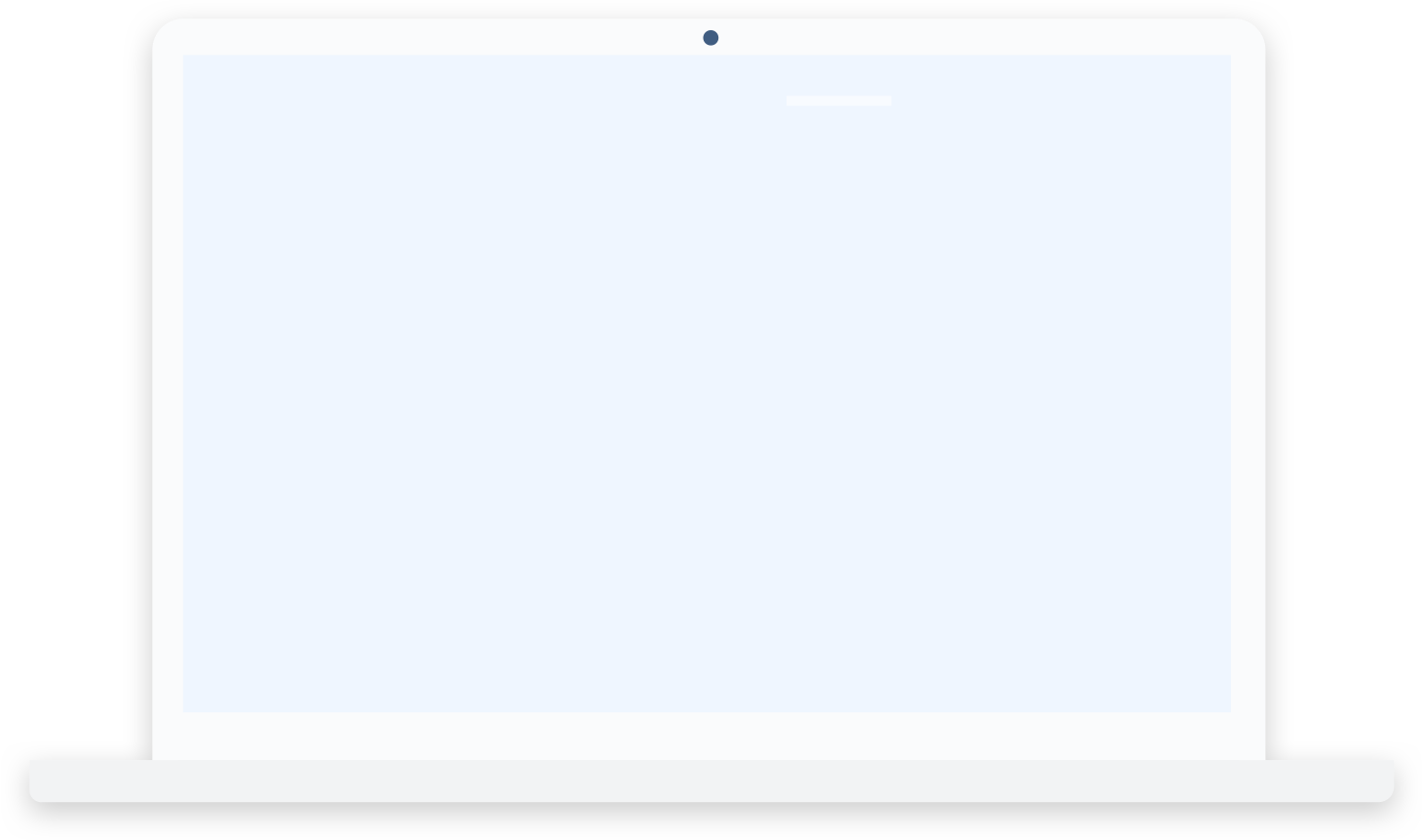The image depicts a laptop computer screen with a distinct white border. The integrated camera is a dark blue dot, positioned centrally at the top edge of the screen. The display itself features a pale blue background, lighter than baby blue, providing a soft, pastel hue. There is white text on the screen, although its content is not legible. Notably, the laptop seems to lack a visible keyboard, suggesting it might be concealed or the image is focused solely on the screen. The overall setup appears to be resting on a flat surface, reinforcing its desktop-like appearance.